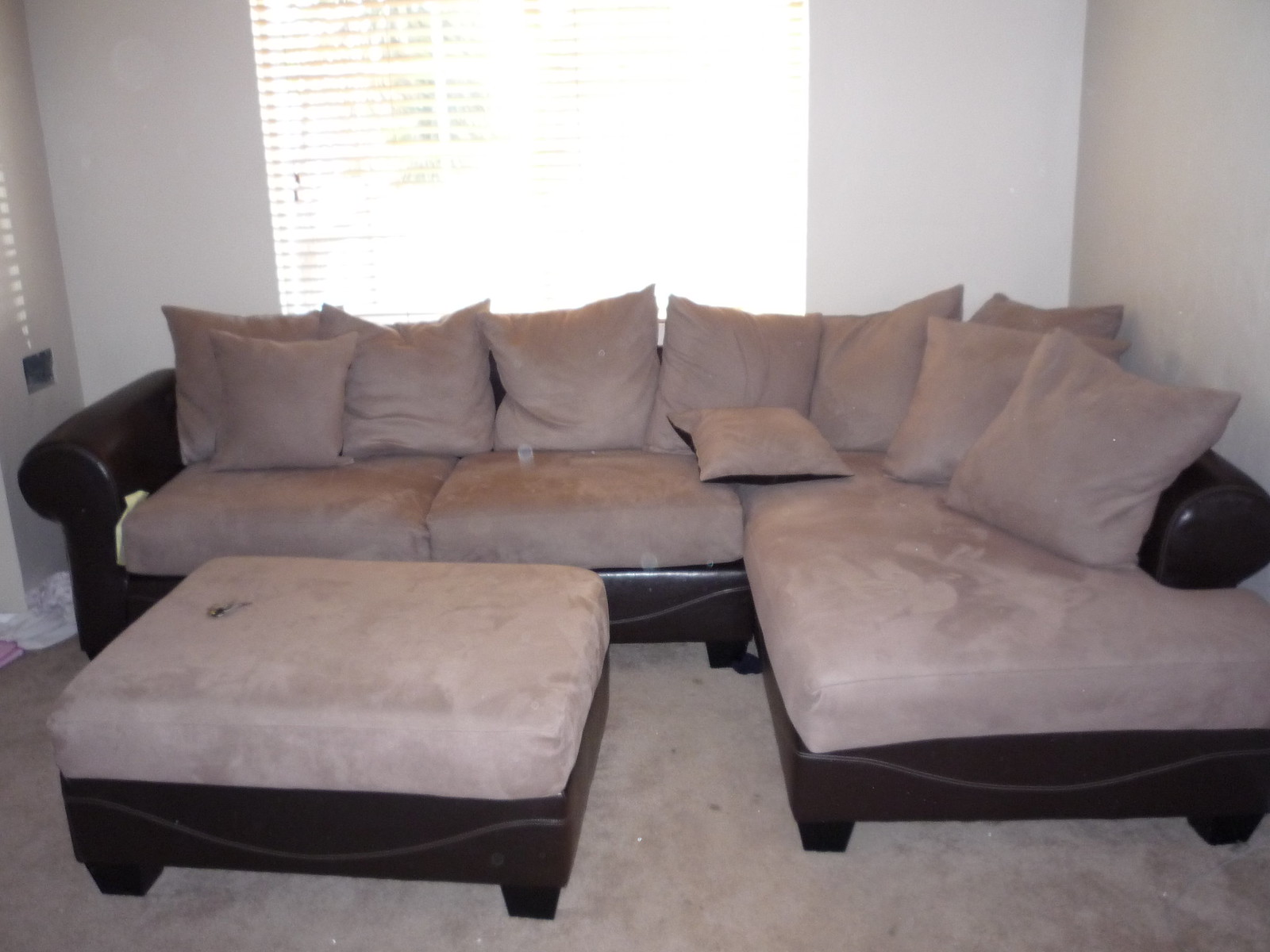The photograph depicts a small, poorly maintained living room in color, likely taken indoors. The bland off-white or cream-colored walls, devoid of any detailed decor, enclose the space. On the left wall, halfway down, there's a mysterious black square, and a large window on the left center of the back wall is inundated with an overwhelming amount of bright white sunlight, filtered through white shades or Venetian blinds.

Dominating the room is a shabby sectional couch with an unappealing mix of materials—its base and arms are covered in an artificial brown leather, while the stained, velvety lighter brown cushions and individual square pillows show signs of neglect. The floor features a close-shaved light gray carpet, which shares in the room’s overall state of dinginess and is mirrored in the color of the couch’s ottoman, centrally placed. Scattered clothing lies in one corner, adding to the overall disheveled appearance.